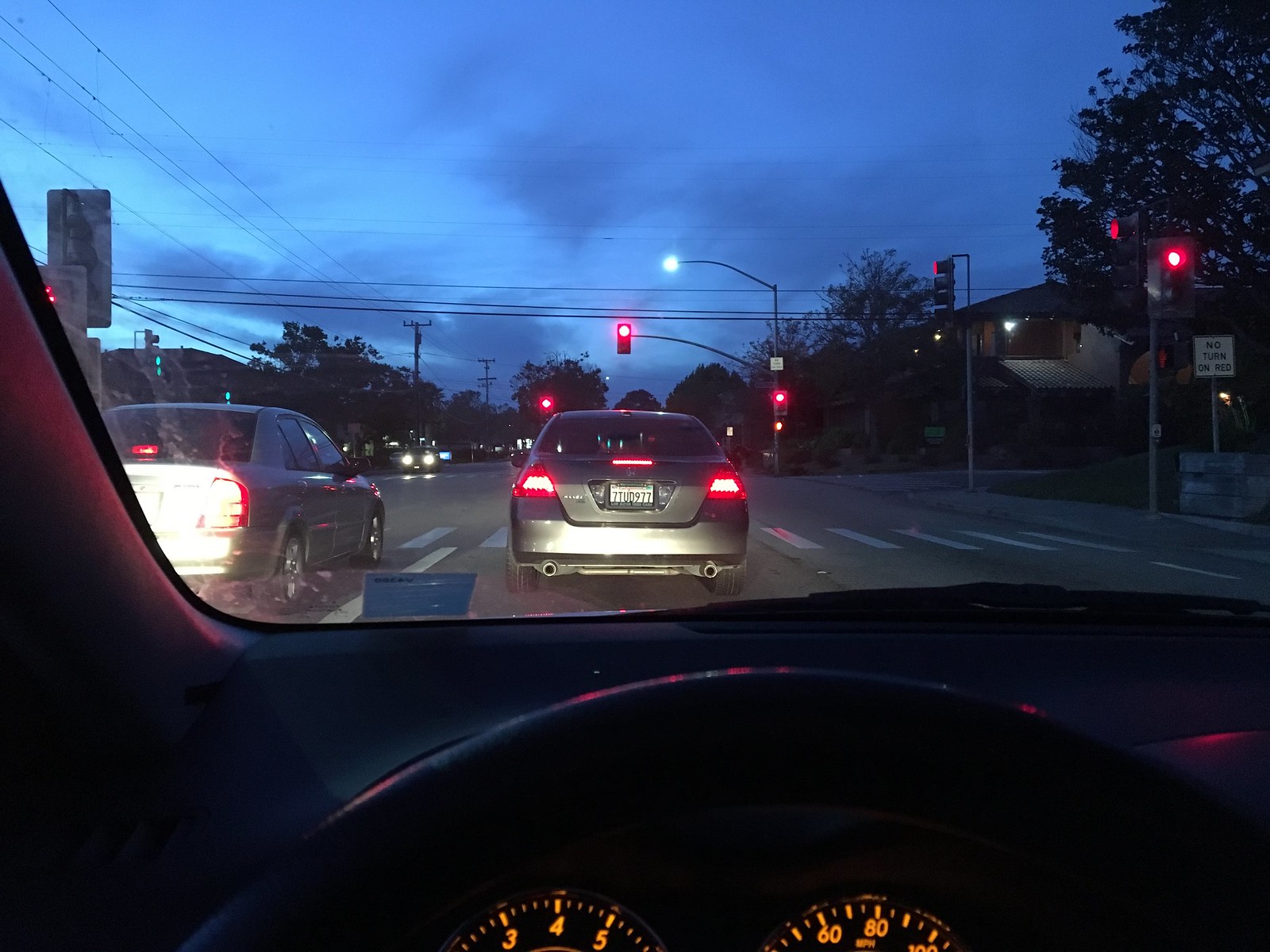This detailed color photograph captures the perspective of a driver sitting behind the wheel, looking out through the windshield as they approach a large intersection. The image, taken either near nightfall or shortly before sunrise, features a cloudy sky with glimpses of blue. Directly ahead, a gray car with its taillights flashing red is stopped at a red light, positioned at a major intersection known from the presence of multiple red traffic lights—three or four are visible—and a street lamp illuminating the scene. Additionally, a vehicle in the left lane, likely bluish-gray in color, is also visible with its lights on. To the right, pedestrian crosswalk lines can be seen clearly. The surroundings suggest an established residential neighborhood with large trees and buildings—possibly apartments on the left and houses on the right. The dashboard of the car from which the photo is taken is partially visible, featuring a couple of analog dials, likely including a speedometer.